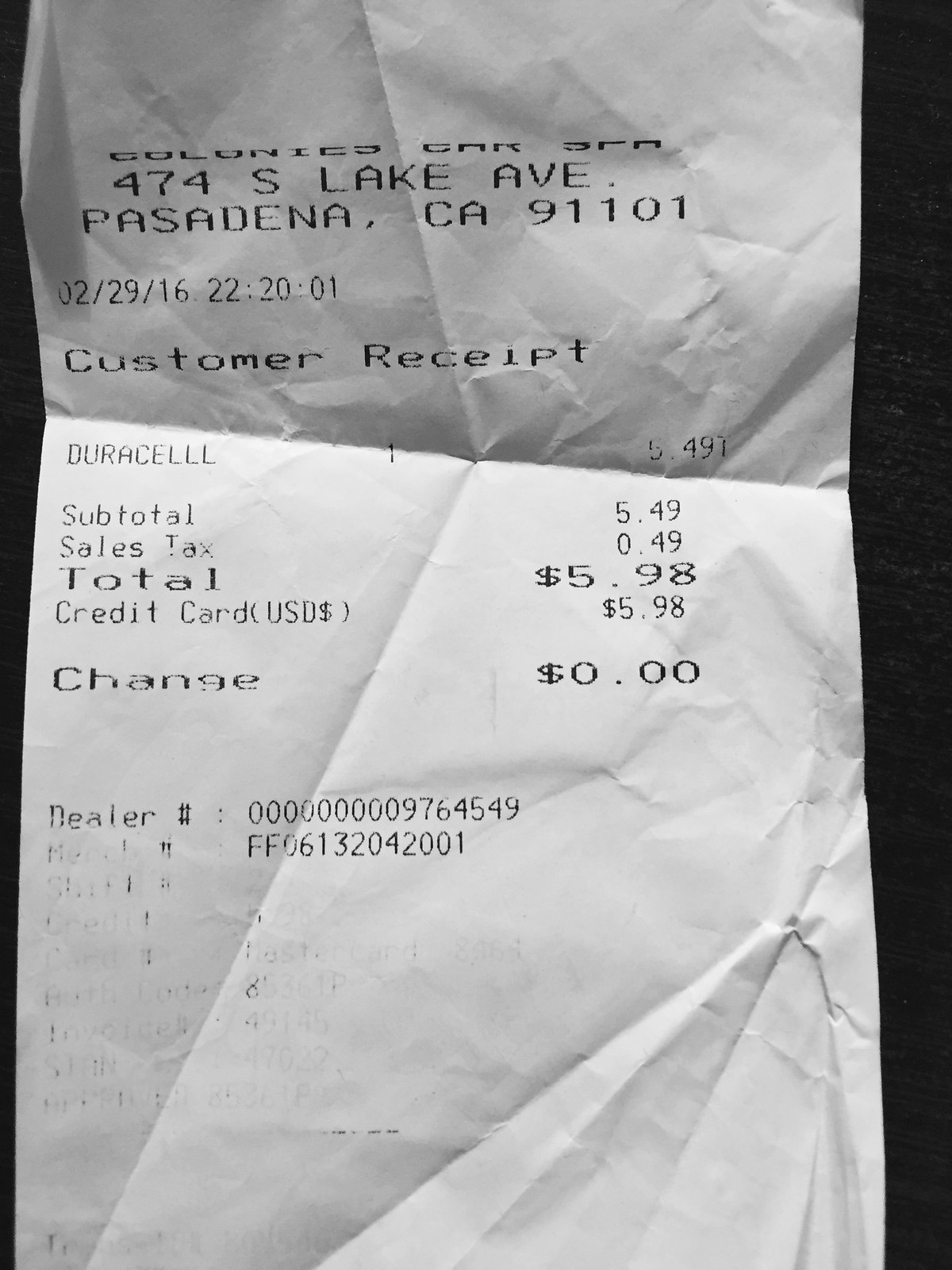This photograph depicts a slightly crumpled and creased white paper receipt set against a black background. The receipt is from Colonies Car Spot located at 474 S. Lake Ave., Pasadena, CA 91101. The purchase was made on 02/29/16 at 22:20:01. This customer receipt details a purchase of a Duracell battery for $5.49. The subtotal of 5.49 is followed by a sales tax of $0.49, bringing the total to $5.98, which was paid via credit card (USD) with no change extended. The dealer number is listed as 00000009764549, with some largely illegible text below it. The receipt is folded both horizontally and vertically, with visible creases and minor crumpling at the edges. Some text near the bottom left is faded and partially obscured.